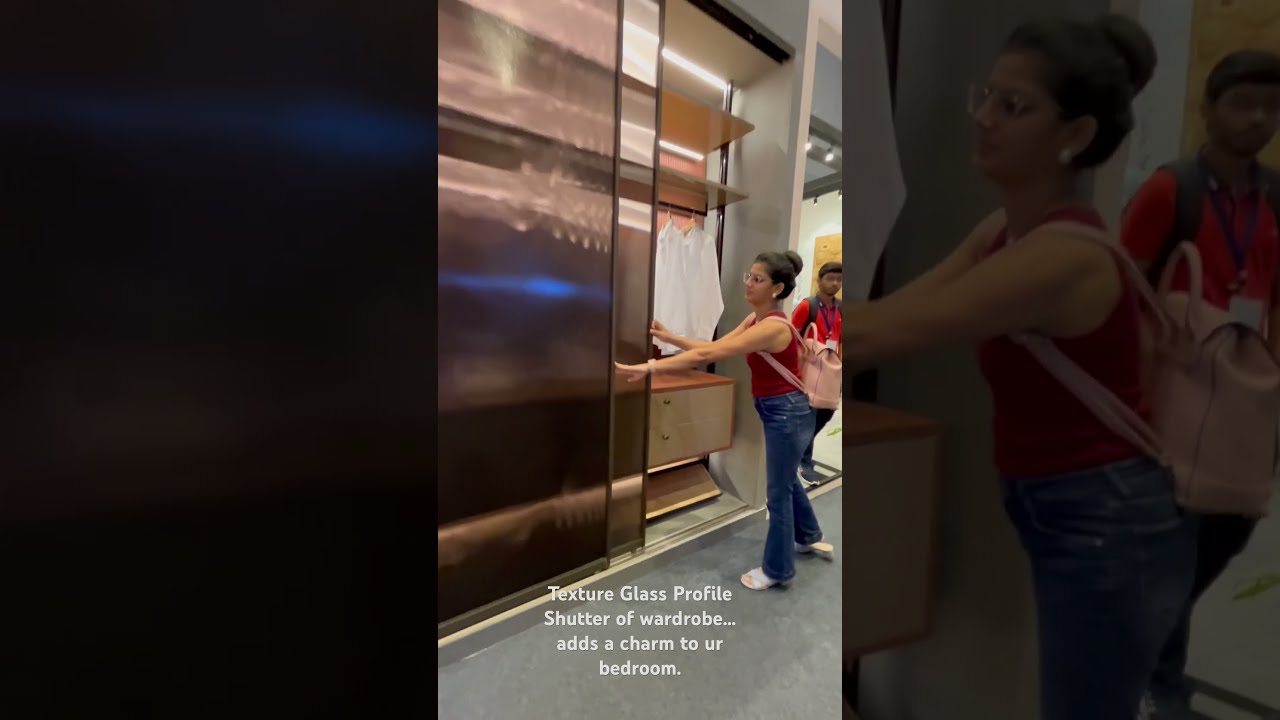In the center of the vertically-aligned, three-panel image, a woman, seemingly of Indian descent, is depicted pushing open a tall, bronze-colored sliding wardrobe door within a brightly lit store. The left panel is almost entirely black, while the right is a translucent, zoomed-in version of the center, both featuring a faded effect. Behind the door, several white shirts hang neatly on rods above a wooden platform with potential drawers or compartments. The woman, wearing jeans, a red tank top, a black cross-body bag, and a watch, stands on a gray concrete floor. Beside her, another individual, also appearing to be Indian, watches her actions, clad in a red shirt and carrying a backpack. Superimposed white text at the bottom of the image reads: "textured glass profile, shutter of wardrobe, adds a charm to UR bedroom."